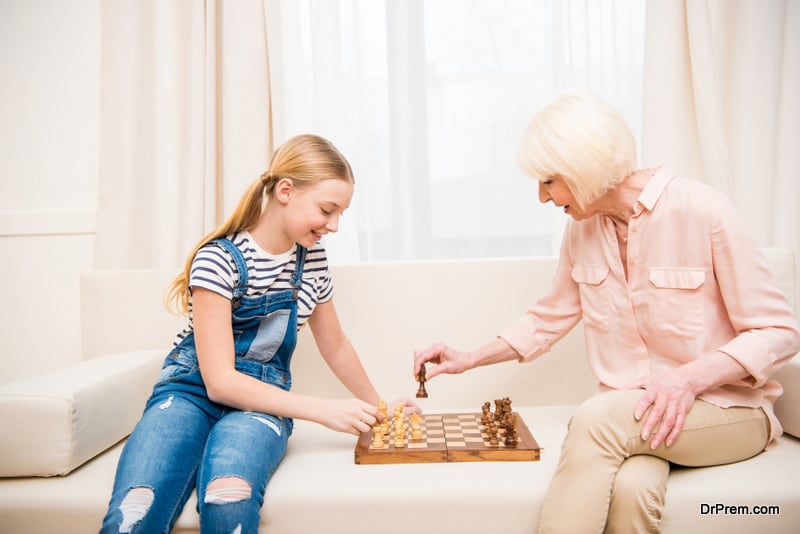In a warm and cozy living room, a grandmother and her granddaughter are engrossed in a game of chess on a beige sofa. The young girl, sitting to the left of the wooden chessboard, has blonde hair styled in pigtails and is dressed in blue overalls over a blue and white striped shirt. She focuses intently, a slight smile playing on her lips, as she moves a chess piece. Opposite her on the right side of the chessboard is her grandmother, an elderly woman with white hair. She is wearing a light pink long-sleeved shirt paired with light beige khaki pants. The room's gentle color palette, including beige walls and light beige curtains framing a window behind them, enhances the scene's serene atmosphere. The wooden chessboard, with its classic light and dark squares, sits prominently between them. In the lower right corner of the image, black text reads "drprem.com," adding a modern touch to this timeless family moment.